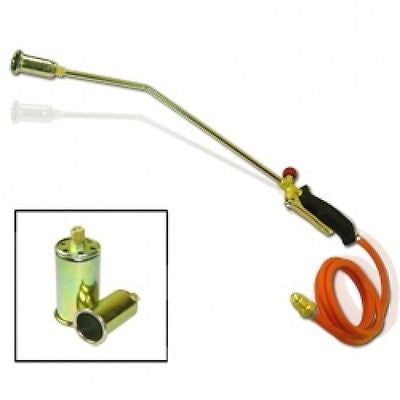The image depicts a low-resolution product photo of a propane torch assembly. The main components include a thick, curled orange hose connected to a black handle via gold metal fittings. This black handle, equipped with a lever-like trigger, supports a bent steel pipe extending towards the top left of the image, culminating in a brass-colored, bell-shaped nozzle. Additionally, the bottom-left corner of the image features a black square inset displaying a close-up of two brassy, cylindrical nozzles, showcasing more detailed views of the fittings and structure at the end of the hose and pipe.